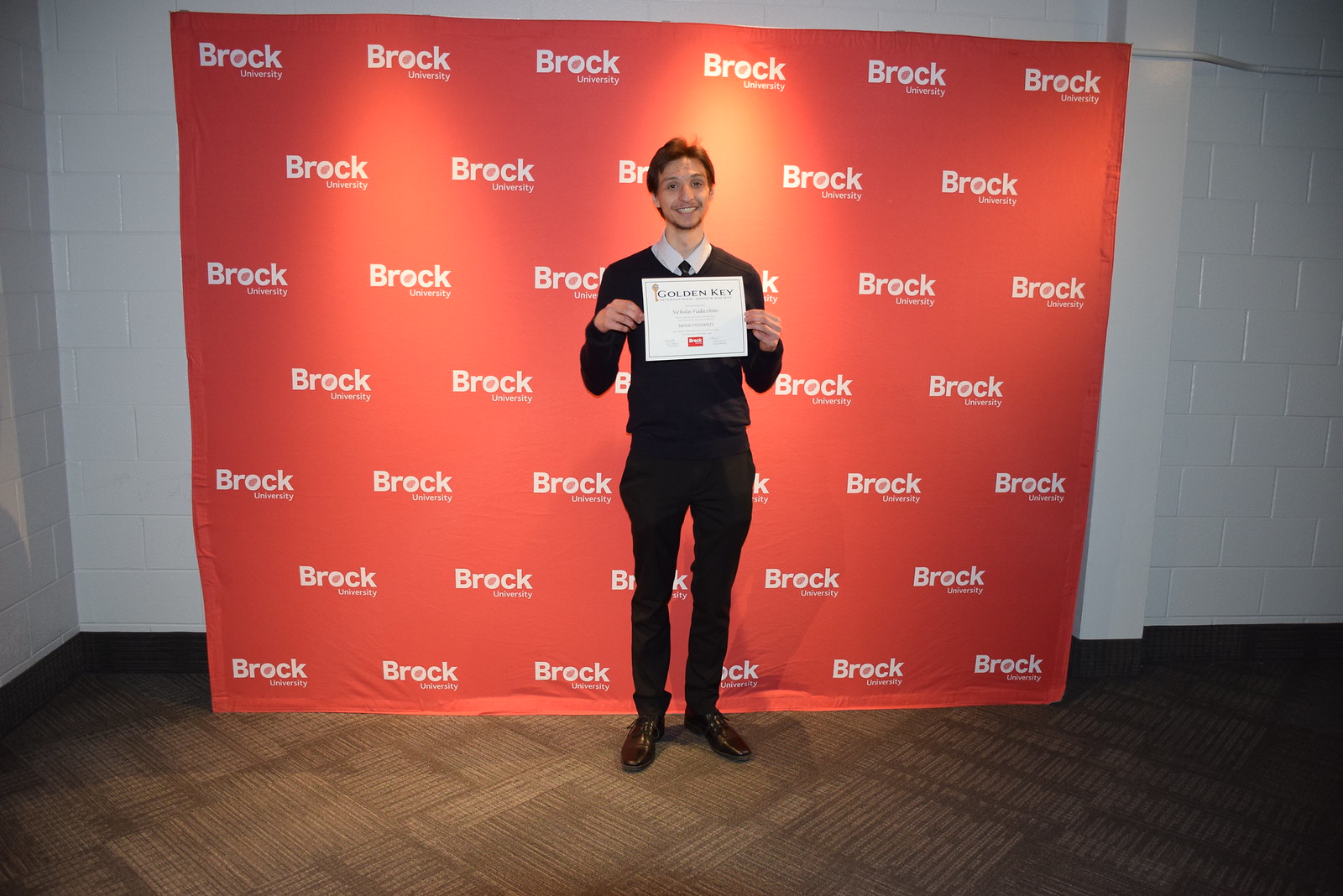A young man in his early 20s, with dark hair and a black beard, stands smiling at the camera in front of an orange banner backdrop that repeatedly says "Brock Company" in white text. He is dressed in a brown long-sleeve sweater over a white business shirt, paired with a black tie, dark brown pants, and shiny brown leather shoes with squared toes. He holds a certificate at chest level, which bears the title "Golden Key" along with additional text underneath. The room features white cinder block walls, and he is standing on a carpet with patterned square sections in shades of tan and brown.